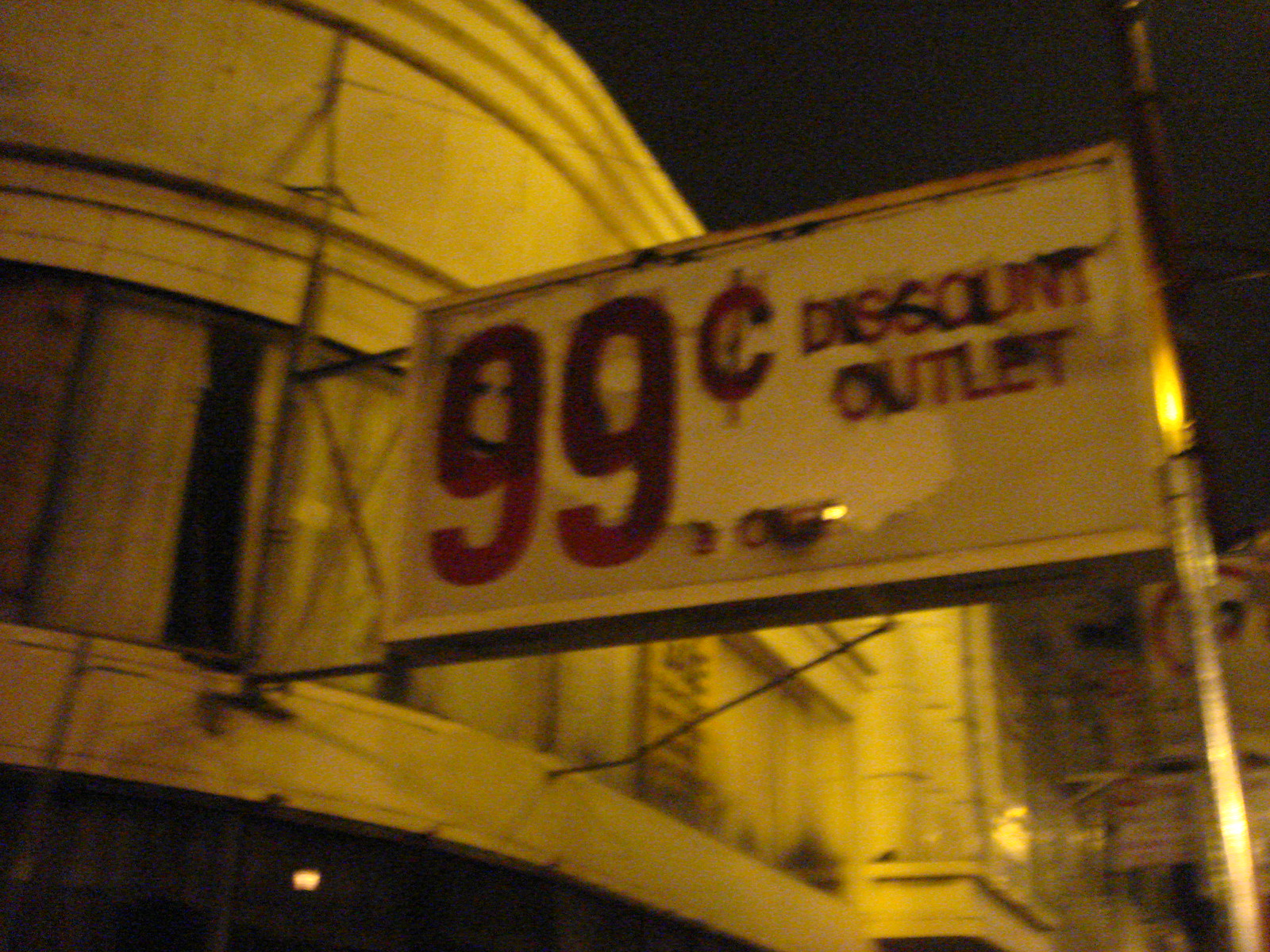This slightly out-of-focus photograph captures a sign prominently attached to a building, positioned centrally within the right half of the frame. The sign, encased in an aluminum frame mounted on an aluminum pole, features large, bold text declaring "99¢" which occupies the left half of the sign. To the right, smaller text reads "Discount Outlet," both elements set against a white backdrop marred by peeling paint.

The sign is bolted to the structure, situated between two windows of the building. Adjacent to the sign, there is a two-story curved building, distinguished by its unique architecture. The background showcases a collection of larger white buildings, adding an urban context to the scene. Additionally, other smaller signs are visible towards the lower right-hand corner of the image, including an unreadable yellow sign seen through a window of the curved building. These elements together create a nuanced portrayal of the locale, highlighting the visual interplay between the sign and its surroundings.